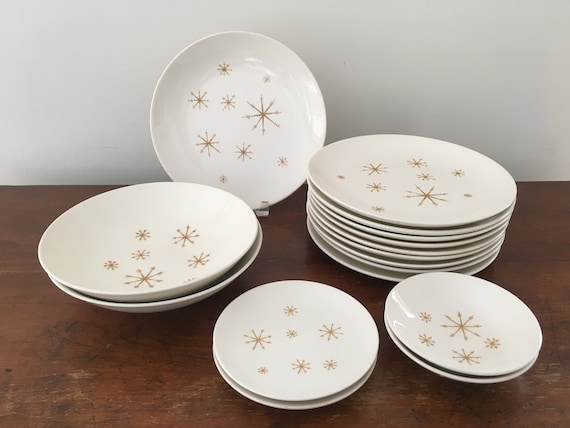The image showcases an assortment of white porcelain dishware with intricate light brown star designs, each star formed by intersecting lines creating an 'X' and a plus sign. These dishes are meticulously arranged on an old, dark wooden table, which is visibly scratched and discolored. In the photograph, we see five distinct stacks: 

- In the middle bottom, there are two small plates stacked together.
- To the right of those, another pair of small plates is stacked.
- Above these, on the middle left, is a stack of shallow wide bowls.
- Further to the right, there is a taller stack of approximately nine large dinner plates.
- Behind these large plates, to the upper left, a single bowl stands vertically, held by a clear display stand.

The detailed setup is against a light blue wall, emphasizing the contrast between the pristine white-and-brown dishware and the aged, dark wooden surface on which they rest.